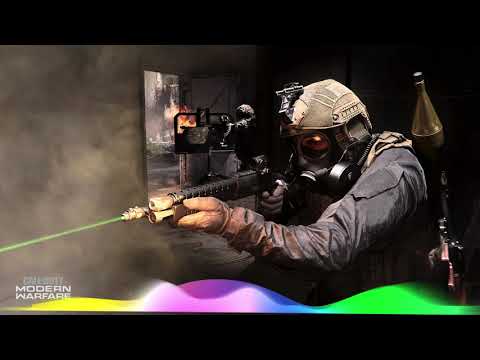This vivid image, likely a screenshot from the hyper-realistic video game Modern Warfare, is framed within a vertically rectangular shape with horizontal black borders, approximately an inch wide, at the top and bottom. The central figure is a soldier dressed in dark shades of brown and gray, adorned with a helmet featuring an attachment and a full-face gas mask, concealing his identity. His attire includes brown gloves and a gray jacket, adding to the rugged look. He is armed with a black shotgun, which extends into a long nozzle equipped with a green laser and a gold tip. The soldier's left arm reaches forward, while his right hand is closer to his body, poised at the trigger. Strapped over his left shoulder is an RPG-style rocket launcher, indicating his heavy combat readiness. The background is a smoky, open area that appears to lead into another outdoor field, with subtle colorful waves from yellow to green suggesting motion or an impending transition. In the image's lower left-hand corner, the game's title "Modern Warfare" is prominently displayed in white, anchoring the dramatic scene.